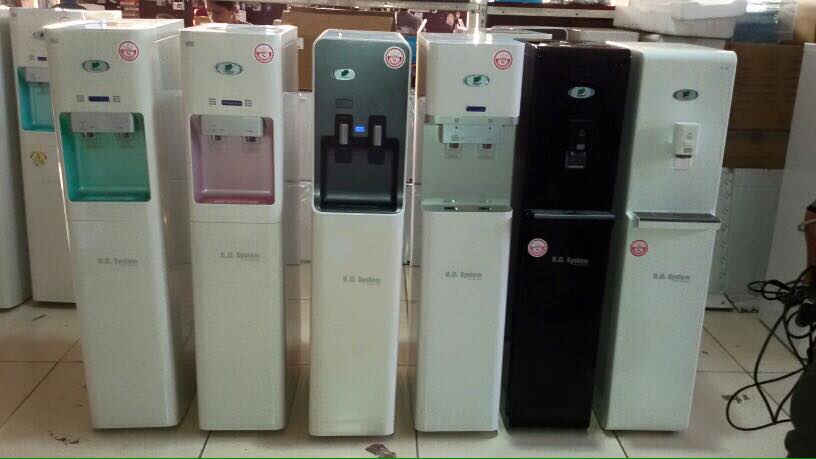The image depicts a row of six standalone water coolers situated on a large white-tiled floor within a warehouse-like environment. The coolers, all of which appear to be of the same brand due to their consistent shape, size, logos, and labels, feature a variety of colors and designs. From left to right:

1. The first cooler is white with a green insert in the dispensing area.
2. The second cooler is also white but sports a pink dispensing area.
3. The third cooler features a white bottom and a black and dark gray top, differing slightly in its water dispensing mechanism.
4. The fourth cooler is entirely white.
5. The fifth cooler is all black and is somewhat hard to see.
6. The sixth cooler is black as well.

Each cooler has a red sticker on the bottom half and a round silver sticker above the handle. Behind the row of coolers, additional appliances, boxes, and other unidentifiable items are visible, reinforcing the warehouse setting. Some electrical cords and a black object are seen in the lower right-hand corner of the image.